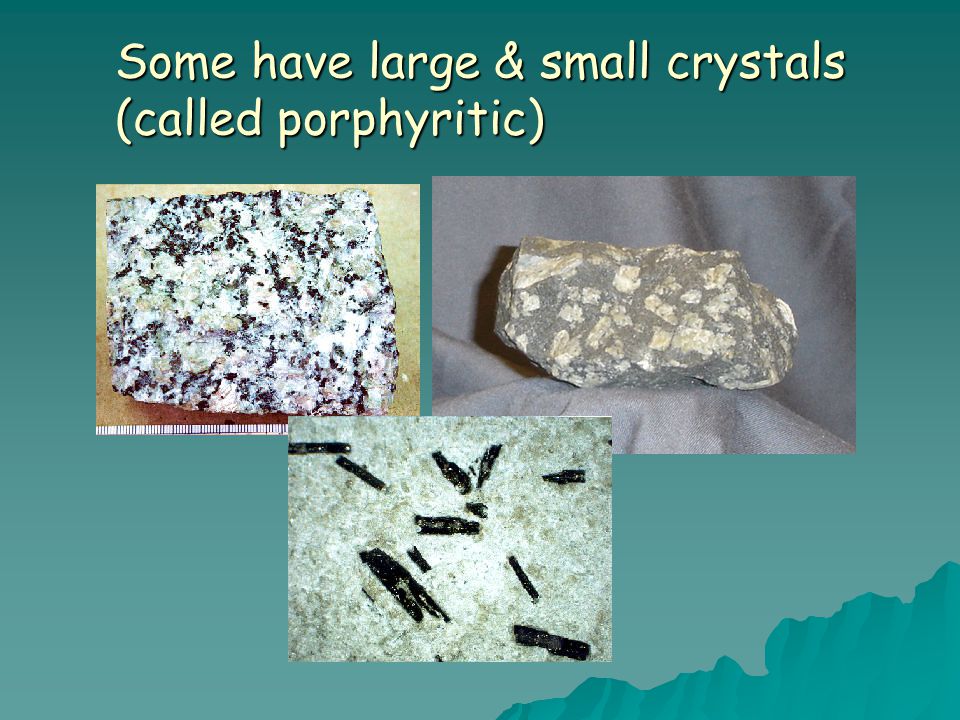The image is a detailed PowerPoint slide adorned with a sea-green, bluish color gradient background, featuring three embedded photographs of various types of rocks and crystals. The slide is topped with a heading in light yellow that reads, "Some have large and small crystals (called porphyritic)." The first photograph, positioned to the top left, showcases a granite-like rock laid against a wooden backdrop. To the top right, the second photo displays a gray stone with white highlights and pinkish speckles, resting on a cloth. The third image, carefully layered over the bottom portions of the first two pictures, is a close-up view of a white and greenish rock with prominent black chips. The arrangement of these images and the descriptive text suggest that the slide is part of a presentation, likely made using PowerPoint, aimed at illustrating different textures and types of crystalline formations in rocks. The background also includes subtle artistic decorations in the bottom right, enhancing the visual appeal.